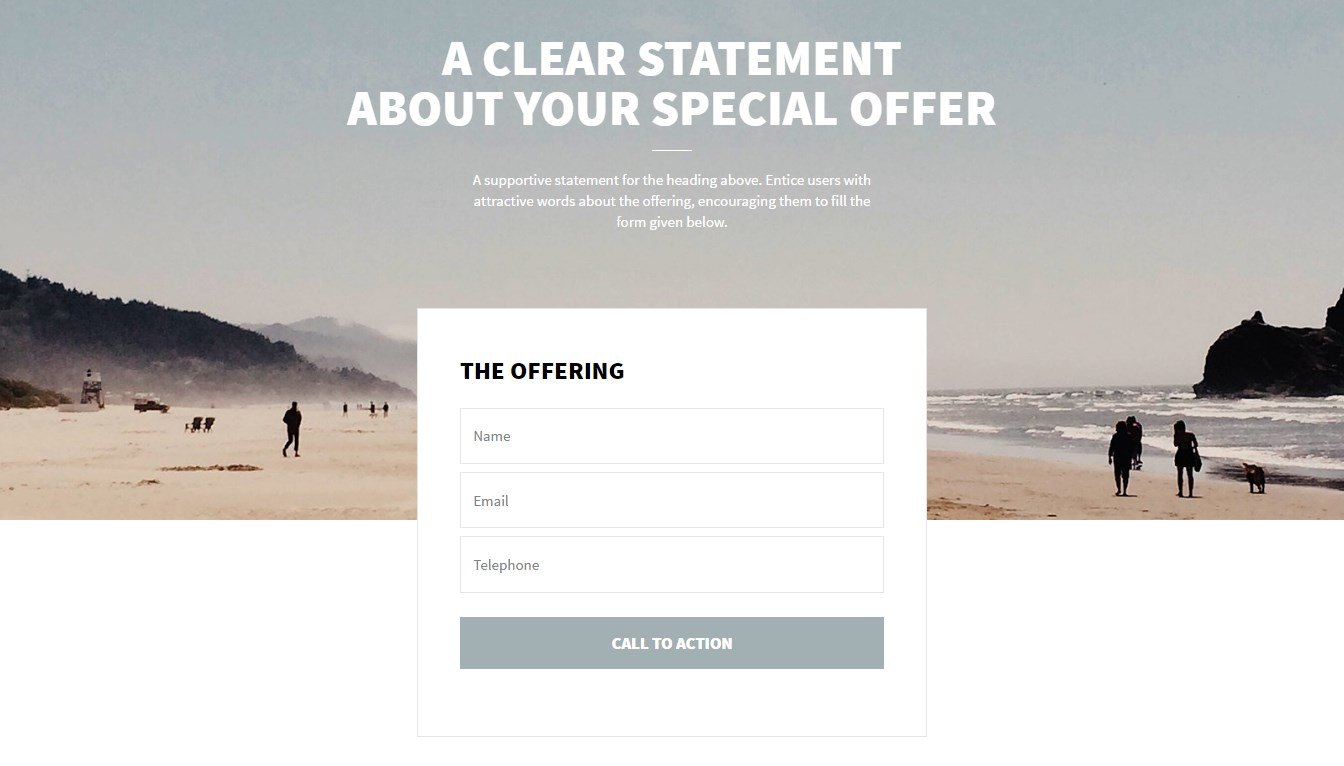The image is a horizontally oriented screenshot showcasing the upper portion of a web page. Dominating the center of this section is a white pop-up box with a thin gray border, providing a clean, minimalistic look. This pop-up box contains a promotional message and a form for user engagement. 

In bold white text at the top of the pop-up box, the headline reads: "A clear statement about your special offer." Beneath this, a smaller white text provides a supportive statement: "A supportive statement for the heading above. Entice users with attractive words about the offering, encouraging them to fill the form given below."

The form within the pop-up is labeled in bold black font as "The Offering." It includes text boxes for the user to input their name, email, and telephone number, followed by a prominent gray call-to-action button designed to encourage user interaction.

The background image visible above the pop-up box is that of a serene sandy beach. The beach, captured in a light brownish hue, features several silhouetted figures strolling along its length, creating a peaceful, timeless scene devoid of detailed features. To the left, a rocky hillside adds texture to the landscape, while to the right, a solitary stone stands in the water. The ocean waves are clearly visible, enhancing the tranquil atmosphere. Overhead, the sky is a hazy gray, completing the subdued, natural color palette of the scene.